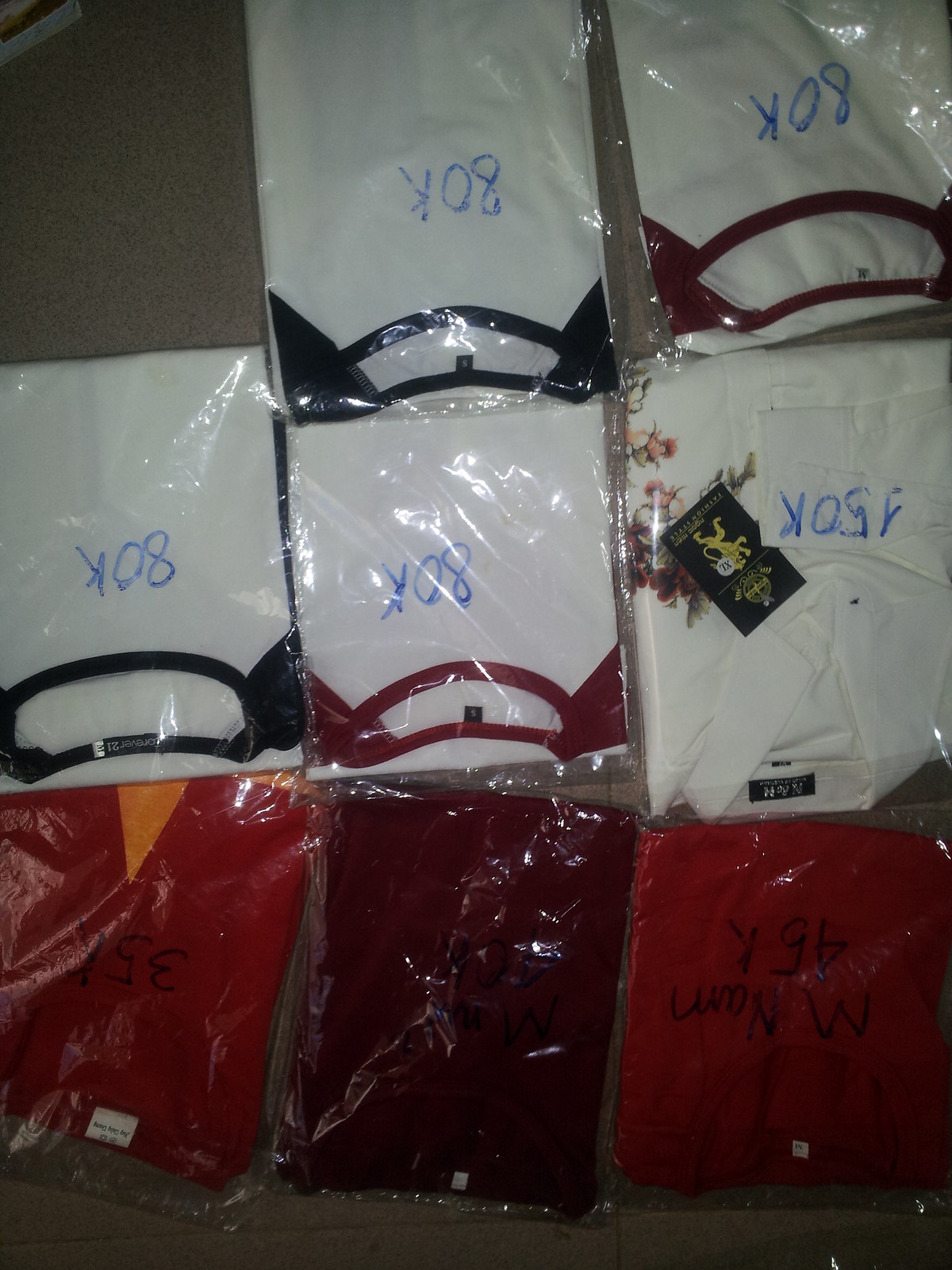The image depicts eight packets of folded t-shirts encased in transparent nylon wrapping, arranged on a grayish-brown surface. The t-shirts are neatly organized in three rows, with the top row containing two packets and the bottom two rows each containing three. The top left corner is notably empty, creating a gap in the arrangement. 

The t-shirts feature a variety of designs, including two solid red shirts, one darker maroon shirt, and five white shirts. Among the white t-shirts, two have black trim, two have red trim, and one showcases a floral pattern. The styles include both round neck raglan sleeves and polo necks.

Each t-shirt has blue marker inscriptions on the front, though the exact details are somewhat unclear due to the dark color of the marker. Five of the shirts appear to bear the number "80K," while another one potentially reads "850K," and one has a mark that resembles "M name 45." The prices or references inscribed range ambiguously from $80K to $95K to $85K, though the exact currency remains unidentified.